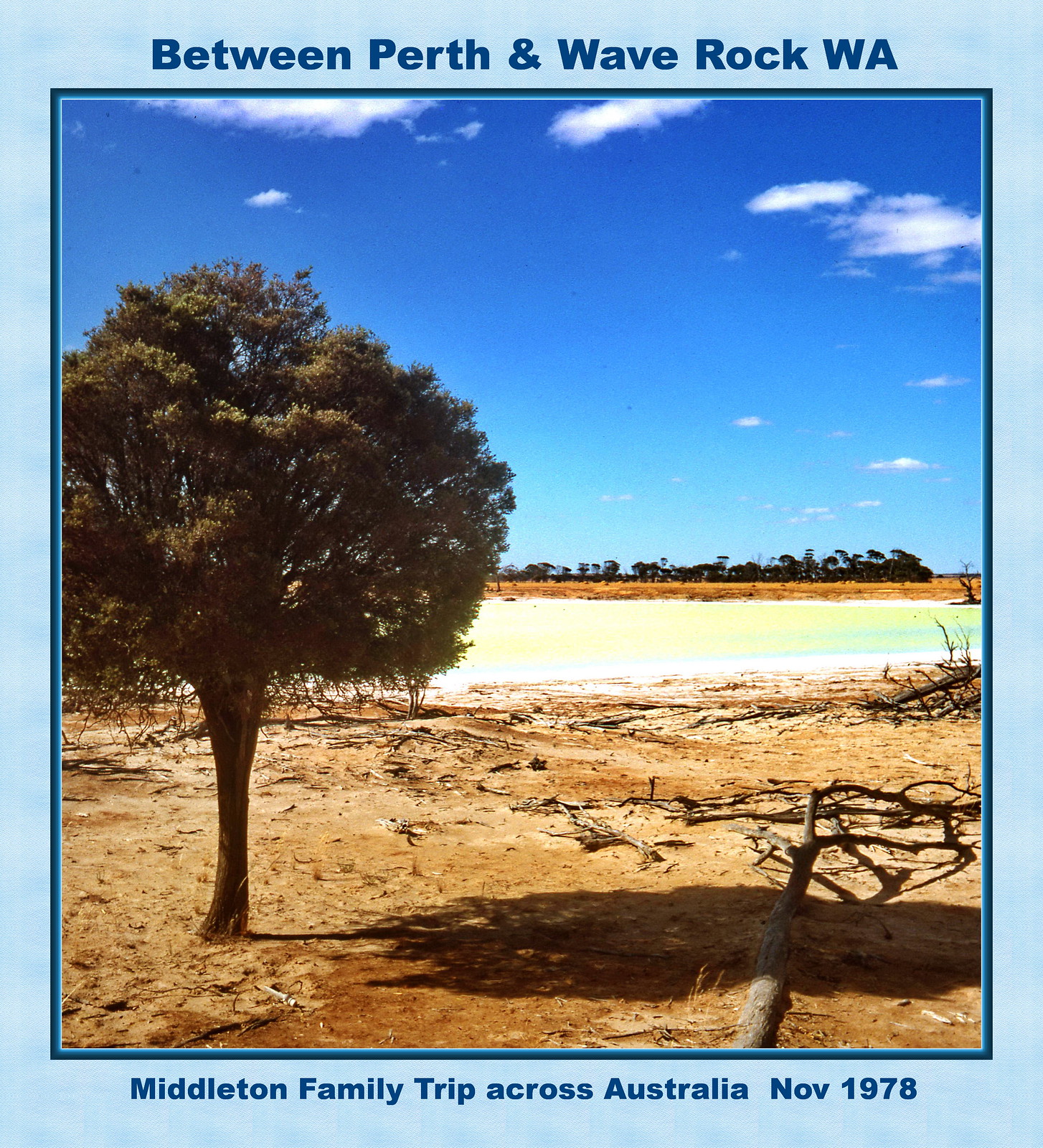The photograph captures a desolate yet striking natural landscape between Perth and Wave Rock, WA, from the Middleton Family Trip Across Australia, November 1978. The primary focus is a short, bushy tree, seemingly parched yet adorned with green leaves, set against a backdrop of hard, clay-like soil interspersed with scattered wooden branches and logs. This desolate area transitions into a dried-out lake bed, distinguishable by its blue and white hues, possibly due to residual salt or sand. Farther beyond, a distant ground area mirrors the foreground with brown soil and clusters of trees. Overarching the scene, a blue sky filled with clouds stretches from the top of the picture to its midpoint. Encasing the photograph is a blue border, inscribed at the top with "Between Perth and Wave Rock, WA" and at the bottom with the trip's label, "Middleton Family Trip Across Australia, November 1978". The colors recorded range from earthy browns and tans to sky blues and sporadic greens, with touches of orange, enhancing the dry, natural essence of the location.